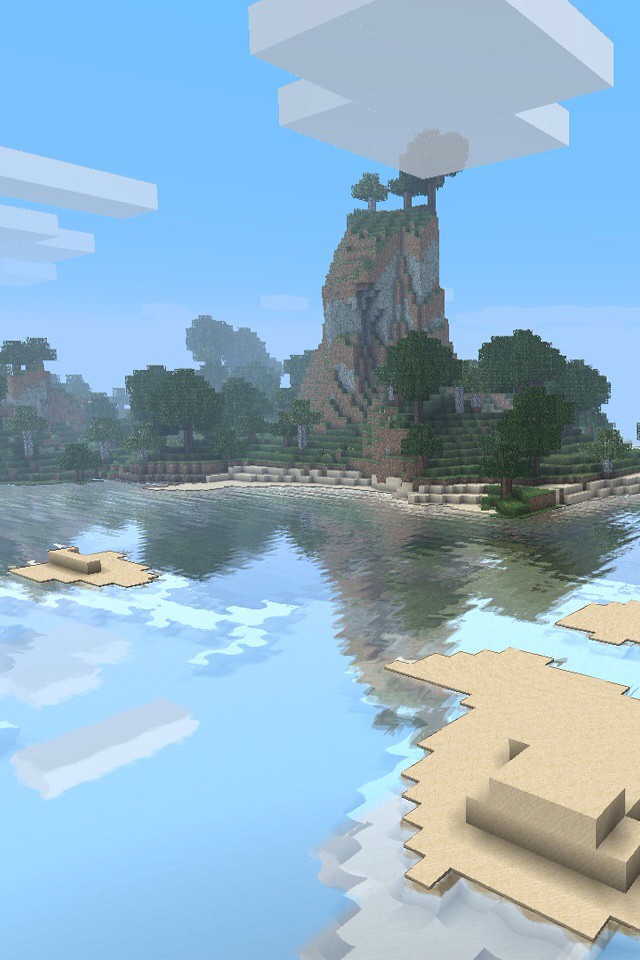This image is a vertical rectangular screenshot from a video game, likely either World of Warcraft or Minecraft. The scene features a mountainous landscape with a cylindrical, trapezoidal mountain in the background. The mountain displays layers of brown and gray rocks, with dark green trees at the top and sides. The image also shows a light blue sky with rectangular, white-accented clouds. Below the mountain, there's a crystal-clear lake that mirrors the mountain, sky, trees, and clouds. The lake has small floating islands or horizontal tan shapes, along with reflections of nearby objects. The area surrounding the lake is lush with greenery, including various green shrubs, grass, and more dark green trees. Some beige and dark brown blocks line the beach area beside the lake, contributing to the overall blocky, low-definition aesthetic resembling an 8-bit style.